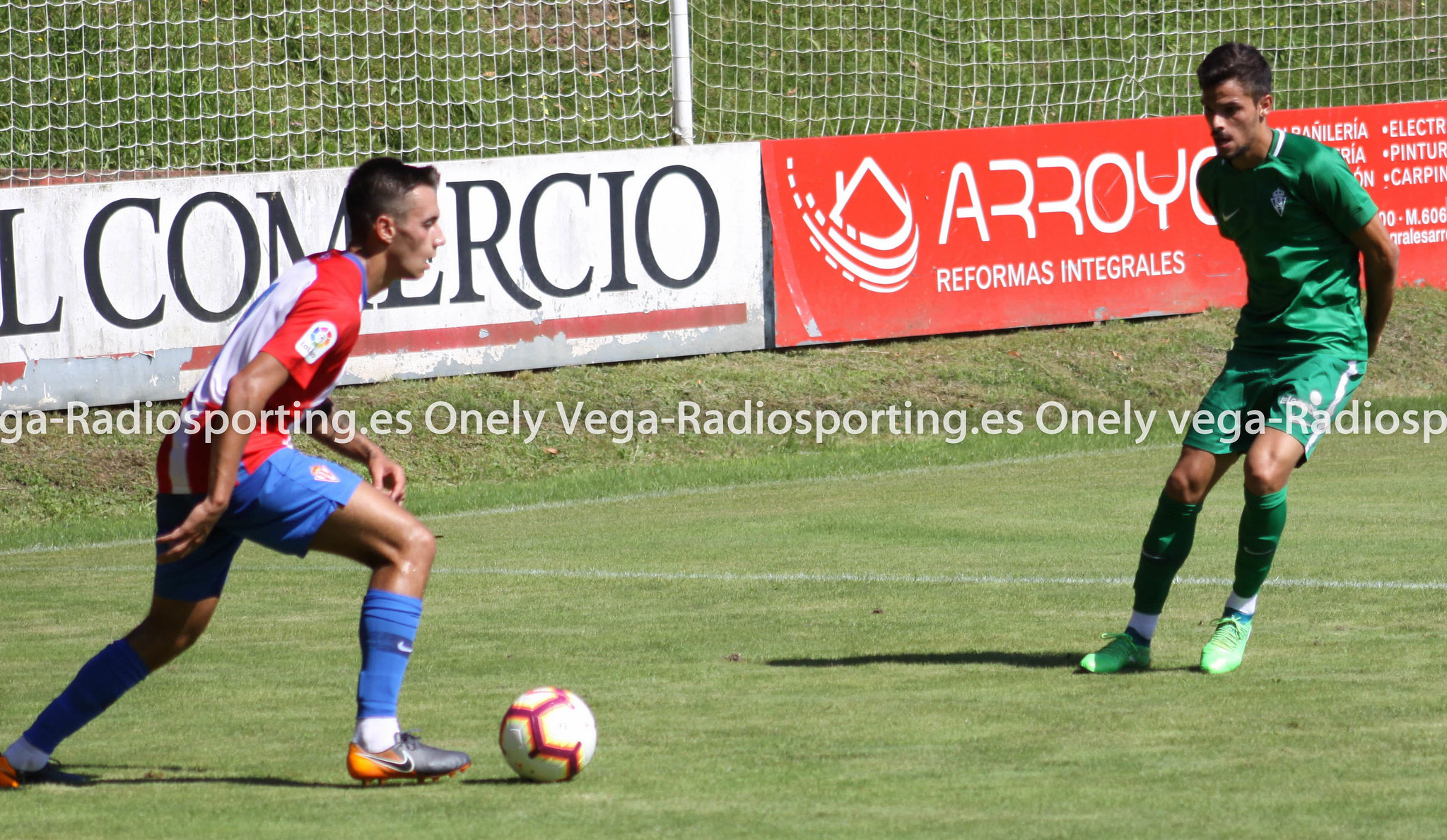In this dynamic image of a soccer match, we see two players in action on a grassy outdoor field marked with white lines. Central to the composition are the players: the one on the left, from the team in red, white, and blue, is about to kick a white soccer ball with red accents. This player sports a red and white top with blue shorts, blue socks, and gray and gold shoes. Opposing him is a player dressed in an all-green uniform with white accents, standing guard with hands behind his back. The backdrop features a green area beyond a white net and various banners, including one that reads "Commercial Arroyo Reformas Integrales." The vivid colors and details indicate a mid-game moment, set under the open sky in the middle of the day.